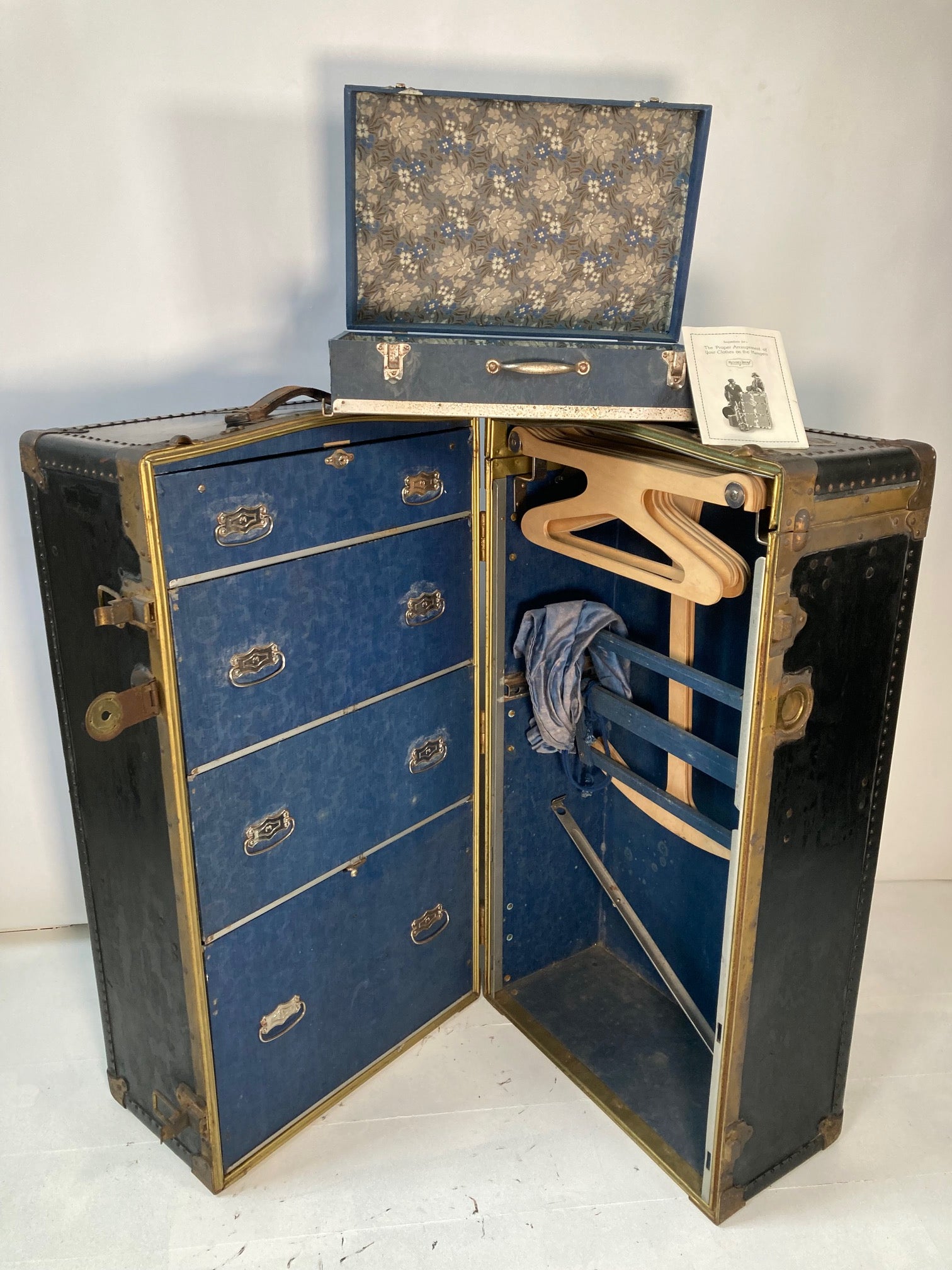The photo depicts a very vintage travel trunk with an exotic hardwood exterior, edged and finished with brass rivets that exude an old-world charm. The trunk, which appears to serve the dual purpose of a portable closet and dresser, is open to reveal two distinct sections. On the left side, there are four drawers designed to store various items neatly. On the right side, built-in hangers offer space to hang clothing, making it a practical storage solution for travelers of ancient times. Above the sectioned trunk sits a smaller suitcase, which is decorated with a floral pattern on the inside of the lid and contains what looks to be an instruction manual. Both the trunk and the suitcase showcase a remarkable level of craftsmanship and attention to detail, highlighting their use in bygone eras for those who needed to transport their personal belongings and maintain organization on the go.